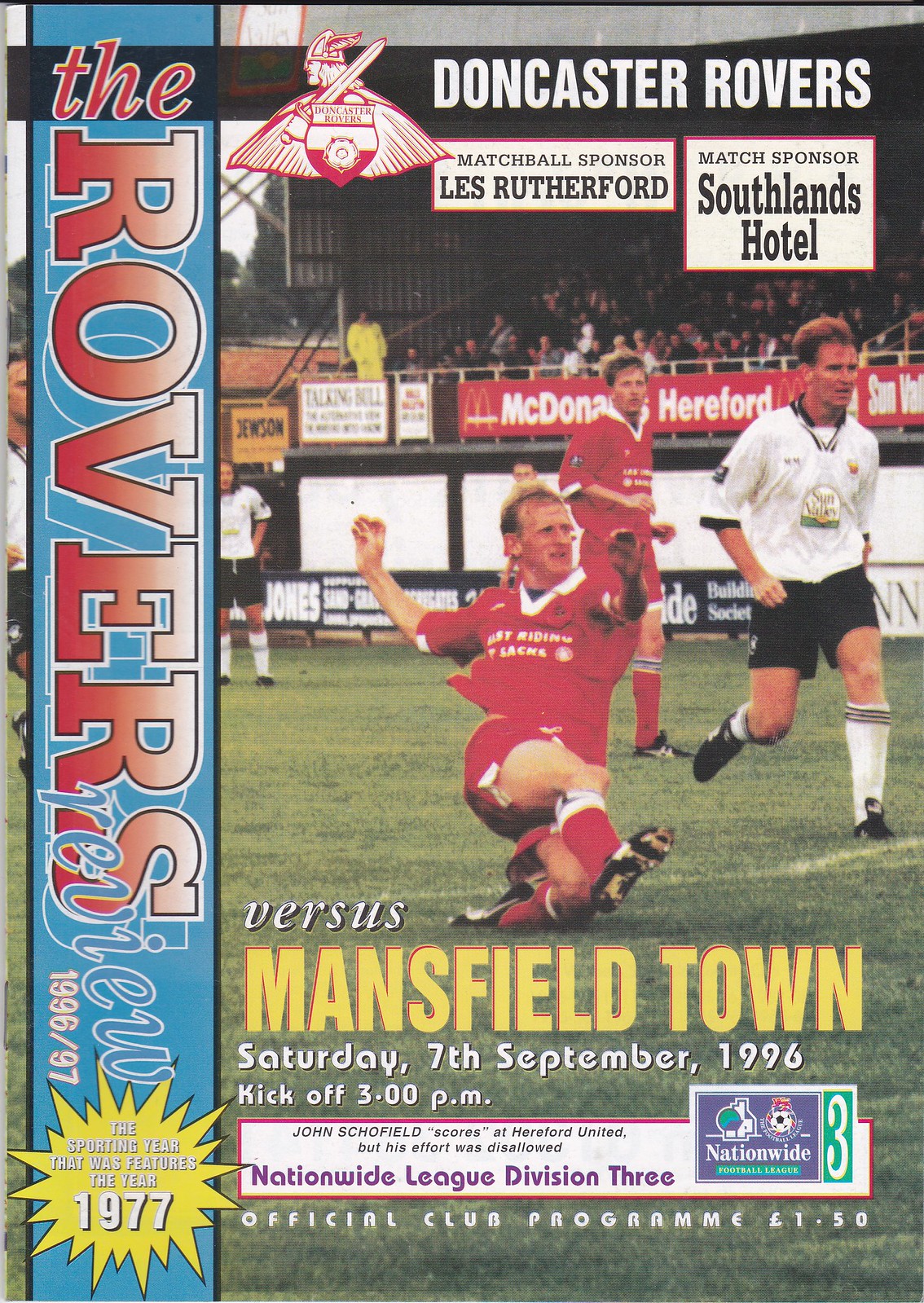The cover of this program for a British football match features an action-packed photo of players competing on a green field. Predominantly on the right side, it showcases two men wearing red shirts and red shorts—presumably from the Doncaster Rovers—alongside two opponents in white t-shirts and black shorts. Dominating the left side is a vertical blue banner, with "The Rovers" written in red letters from top to bottom and "Review" in blue letters at the bottom, highlighting the magazine's name. The year "1996-97" is prominently featured in white letters. Additionally, a yellow sunburst with white letters displays "1977" in larger text.

At the top of the cover, a black banner contrasts with the white text "Doncaster Rovers," accompanied by their logo of a Viking character with a sword, shield, and wings. The detail "Mansfield Town" indicates their opponent, and further down in yellow text, it notes the match date and time: "Saturday, September 7th, 1996, kickoff at 3 PM." The background includes sponsor logos on the stands, and it’s indicated that this is the official program with a price of 150 pounds.